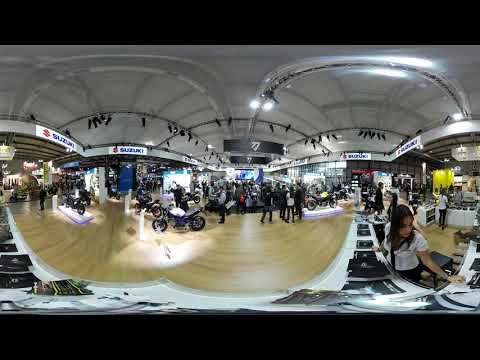This image captures a bustling indoor Suzuki motorcycle convention, likely held in a large hall with parquet wooden flooring. The photograph appears to be taken in a panoramic format, causing some distortion, particularly around the edges. In the foreground, a long table laden with several closed laptops can be seen, with a woman seated at one end, possibly interacting with attendees or working on something just off-frame. In front of her lies an assortment of brochures. 

Signs emblazoned with the Suzuki logo are prominently displayed near the ceiling, confirming the brand focus of the event. Track lighting is installed overhead, which, along with various exhibit lights, brightly illuminates the interior. The middle ground is dominated by numerous motorcycles, drawing the attention of the vast crowd present. Attendees can be seen walking and gathering around the bikes, exploring the different models on display. Overall, the lively scene suggests a well-attended event dedicated to showcasing Suzuki motorcycles and related products.